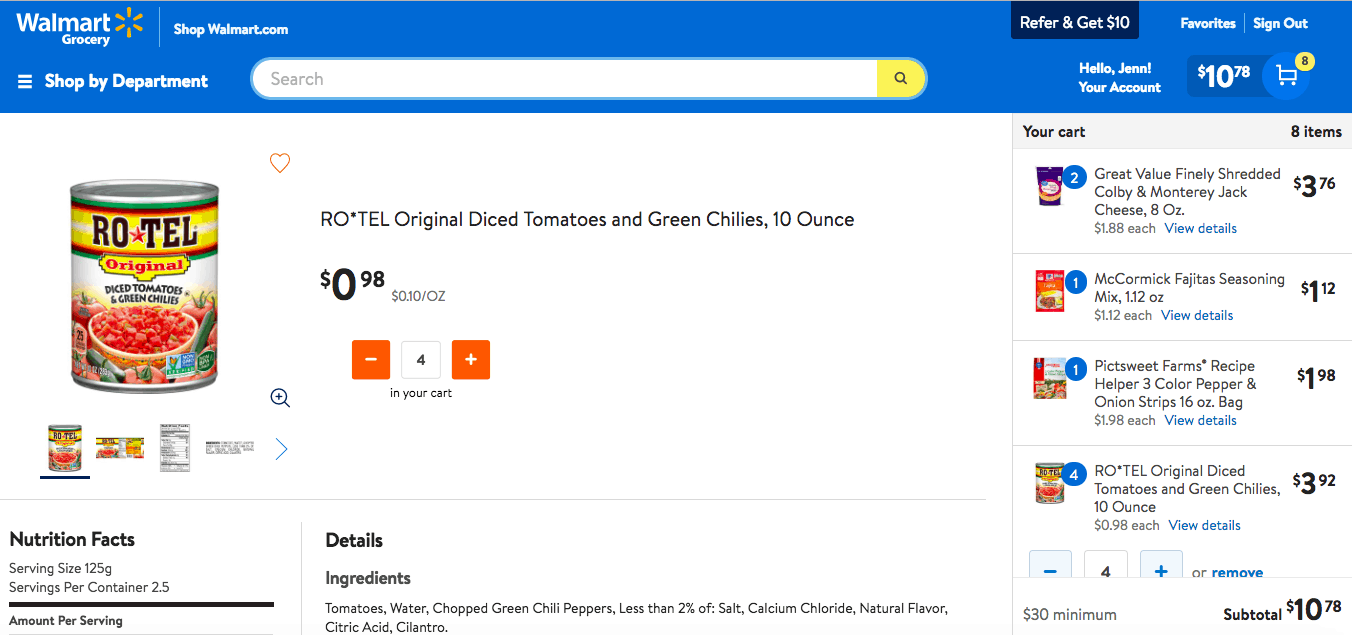The image depicts the Walmart Grocery website. In the upper left corner, the words "Walmart Grocery" are prominently displayed alongside the iconic yellow Walmart asterisk logo. Adjacent to this is a banner ad promoting ShopWalmart.com, with a black box within the ad that offers a referral deal: "Refer and get $10."

Below the banner, a greeting reads, "Hello Jen," indicating the account holder's name. Jen's account details are visible, showing her cart with 8 items totaling $10.78. Jen is currently viewing a product page for canned Rotel. The page includes a main image of a can of Rotel, accompanied by smaller thumbnails below, which provide detailed information such as nutritional facts and ingredients.

Jen has selected 4 cans of Rotel, though she has not yet added them to her cart. The rest of the webpage displays the contents of her cart and additional details about the Rotel product.